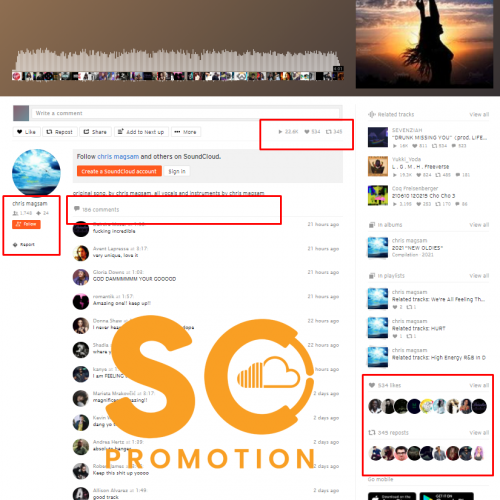This detailed descriptive caption provides an extensive overview of a SoundCloud page screenshot viewed on a desktop website.

The top section of the image showcases a brown gradient background, which serves as a backdrop for a white and gray sound waveform. Running across the entire width of this waveform is a line of square profile pictures.

Adjacent to this on the right, the photograph captures a silhouette of a woman joyfully leaping into the air against an orange, sunlit sky. Above her are a few gray clouds, and below is a dark silhouetted landscape.

Beneath these elements is the primary body of the website, set against a white background. Multiple sections are highlighted with red boxes, drawing attention to specific portions of the page.

Starting from the left, the first red boxed area contains the artist's title, "Chris Magsum," displayed in medium gray text. Below the name are some medium gray icons, accompanied by an orange "Follow" button featuring a white profile icon and white text. Further down, separated by some whitespace, is the dark gray word "Report."

Above this section is a circular profile picture depicting a blue, cloudy sky.

To the right of this initial red box is another highlighted area displaying light gray text that reads "188 Comments," situated next to a gray speech bubble icon.

Slightly higher and further to the right, another red box encapsulates more medium gray icons and text. This includes a triangle with partially visible text, "22 point something," a gray heart icon with the number "534" beside it, and a gray circular arrow icon with the number "345" positioned to its right.

This caption thoroughly describes the visual elements and layout presented in the screenshot.